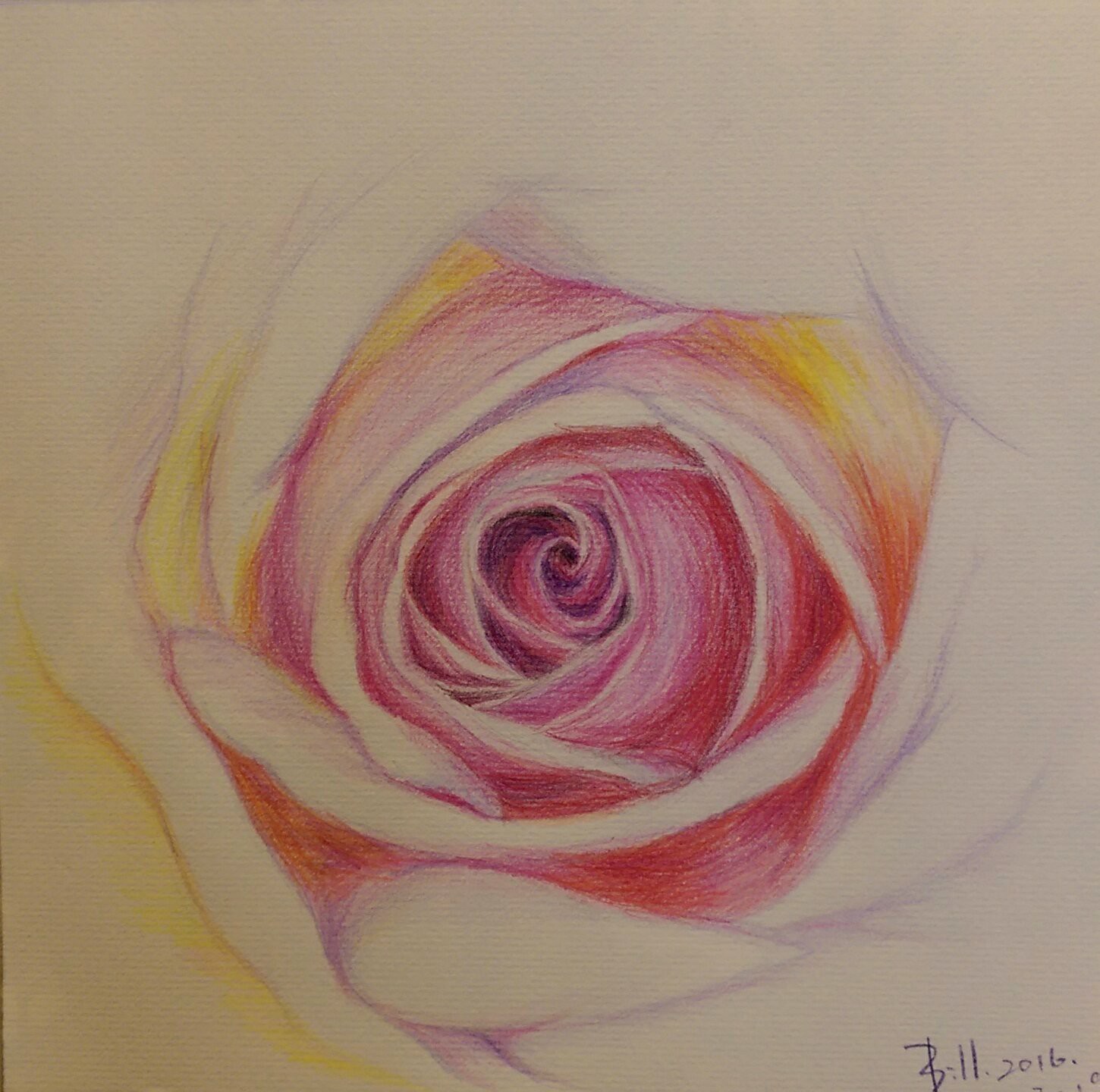This is an intricately detailed colored pencil drawing of a rose, showcasing a vivid array of colors and depth. The drawing focuses on a close-up view of the rose’s center, which is a bright pink, gradually transitioning into deeper reds. The petals spiral outward in a counterclockwise fashion, with their colors transitioning to lighter pinks, whites, and hints of yellow as they extend to the outer edges. The artist has expertly used fine lines to create a realistic texture and depth, making the viewer feel as though they are peering deep into the rose. In the bottom right corner, the artist has signed the piece with "Bill 2016" in bluish ink. This signature partially cuts off at the edge of the drawing, adding a personal touch to the artwork.